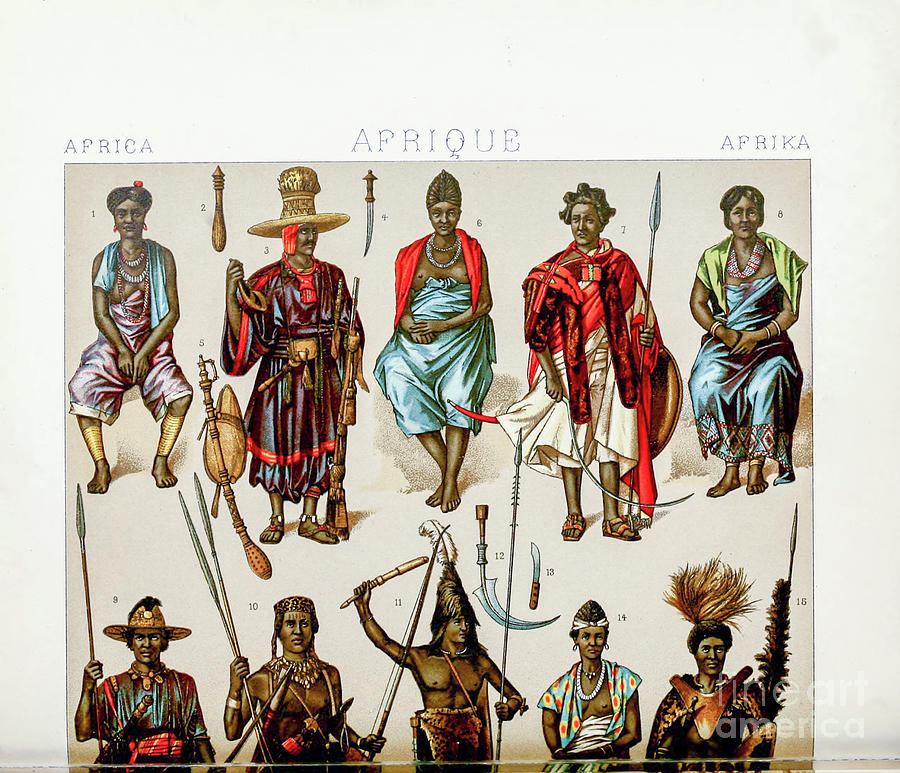This image is an intricately detailed illustration resembling a cartoon or artistic representation that captures various aspects of ancient African culture. In the upper left corner, the title "Afrike" is prominently displayed, spelled "A-F-R-I-Q-U-E." The artwork showcases numerous figures, both male and female, many of whom appear to be members of different tribes donned in traditional attire. For instance, some women are depicted in vibrant blue gowns and red scarves, while a man sporting a black mustache is shown in a distinctive robe.

The illustration includes a numbered key, spanning from 1 to 15, correlating to various items and weapons depicted throughout the scene, such as knives, spears, and even a gun. These items likely represent the tools and weaponry used by the depicted warriors, highlighting their different fighting styles and cultural significance. The artistic portrayal aims to provide a visual representation of the diverse attire, items, and characteristics of people from ancient Africa, offering a detailed glimpse into their historical and cultural heritage.